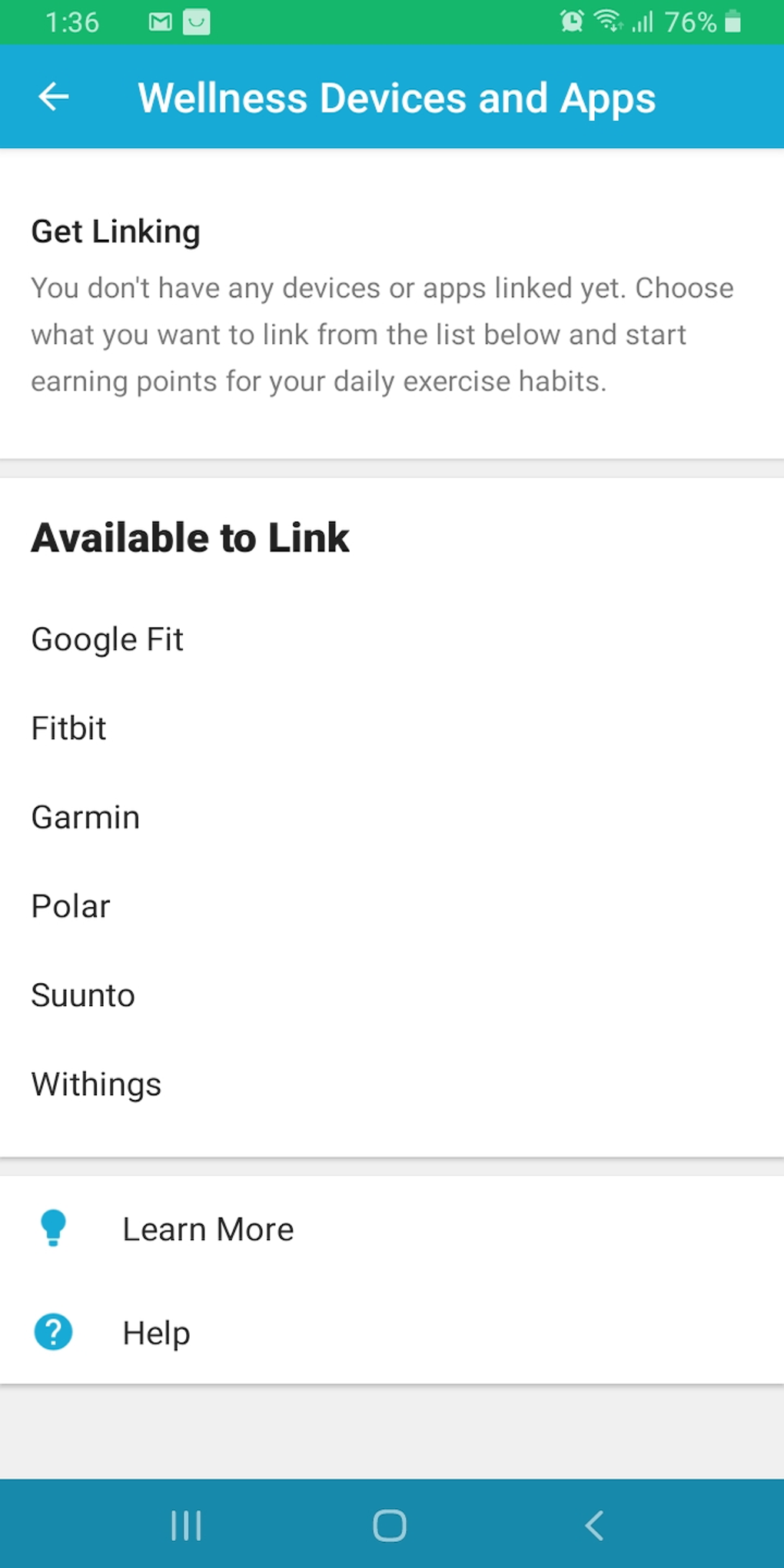The image appears to be a screenshot from a mobile device. At the top of the screen, there is a green status bar displaying the current time as 1:36, a square symbol with an "M" indicating an email notification, a smiley face icon, an alarm clock, a Wi-Fi symbol, signal strength bars, and a battery indicator showing 76% battery life.

Below the status bar, there is a blue rectangular banner featuring a white left-pointing arrow and the text "Wellness Devices and Apps."

Underneath this banner, there is black text that reads: "Get linking. You don't have any devices or apps linked yet. Choose what you want to link from the list below and start earning points for your daily exercise habits." 

The list of available devices and apps to link includes Google Fit, Fitbit, Garmin, Polar, Suunto, and Withings.

Towards the bottom of the screen, there is a blue light bulb icon accompanied by the text "Learn more," and a blue circular icon with a question mark inside, labeled "Help."

At the very bottom of the screen, there is a bluish rectangle that contains three vertical white lines on the left, a white square shape in the center, and an arrowhead pointing to the left on the right.